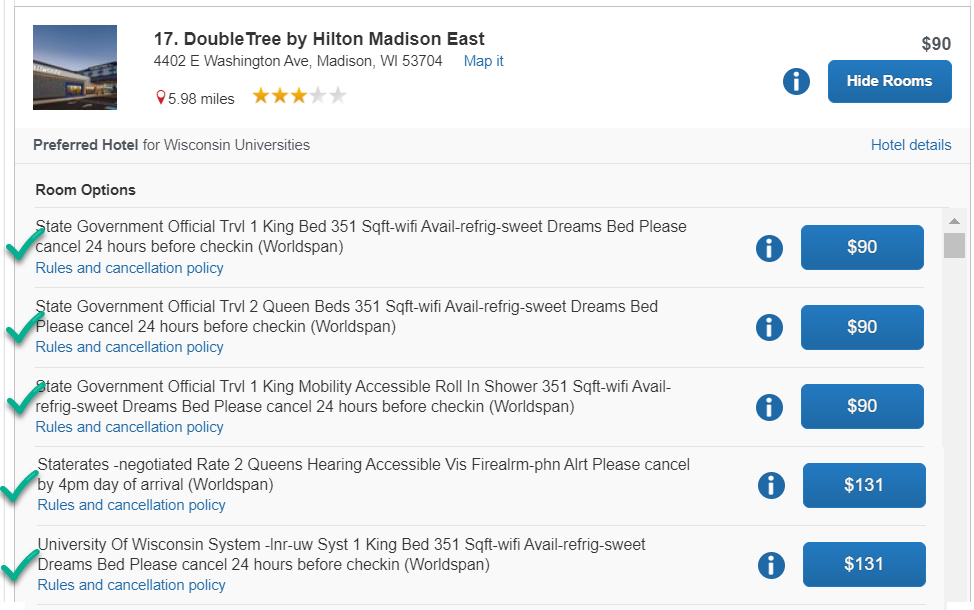**Screenshot Description: Detailed Hotel Information for DoubleTree by Hilton Madison East**

The screenshot features a detailed listing of DoubleTree by Hilton Madison East, showing various information and room options. The background of the screenshot is a light gray, and the content is neatly structured within a box bordered by a gray outline.

- **Header:** 
  - "Number 17" indicates the listing rank.
  - **Hotel Name and Address:** DoubleTree by Hilton Madison East, located at 4402 East Washington Avenue, Madison, Wisconsin, 53704.
  - **Thumbnail Image:** A small square picture of the hotel.
  - **Map Link:** A blue hyperlink text "Map it" which likely opens the location on a map application.
  - **Distance:** Shown in red text, "75.98 miles" from a reference point.
  - **Rating and Price:** Three stars, "75",  and "$90" displayed prominently above a blue "Information" circle with an 'i' and a blue "Hide Rooms" rectangle button.

- **Highlighted Note:** 
  - Displayed on a gray background, "Preferred hotel for Wisconsin universities."

- **Section Titles and Details:**
  - **Room Options:**
    - **State Government Official Travel:**
      - *One King Bed:* 351 square feet, features include WiFi, refrigerator, Sweet Dreams bed. Cancellation requires 24-hour notice prior to check-in. Displayed price is $90.
      - *Two Queen Beds:* 351 square feet, same amenities and cancellation policy as above. Price is also $90.
      - *One King Mobility Accessible Roll-In Shower:* 351 square feet, includes WiFi, refrigerator, Sweet Dreams bed. Follows same cancellation policy with a price of $90.
    - **Negotiated State Rates:**
      - *Two Queens, Hearing Accessible (VIS, firearm, PHN, AIRT):* Cancellation allowed until 4 p.m. on the day of arrival. Price is $131.
    - **University of Wisconsin System:**
      - *LNRUW System, One King Bed:* 351 square feet, offers WiFi, refrigerator, Sweet Dreams bed. Cancellation policy, $131 price tag.

Each section containing room details is accompanied by a blue information icon (i) and the room rate displayed either as $90 or $131 in bold text. Additional specifics include world span codes, rules, and cancellation policies listed under each room option.